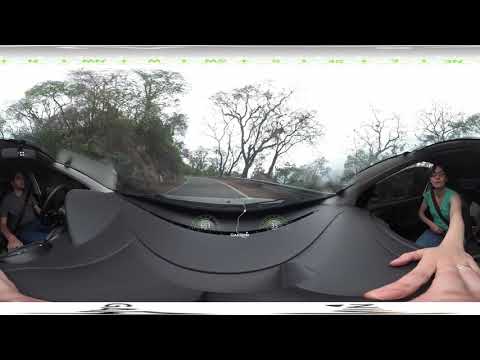This image captures a 360-degree panoramic view inside a vehicle driving along a one-lane road that curves through a mountainous, forested area. The exterior, visible through the curved windshield, reveals large trees with varying amounts of foliage against a hilly landscape. Inside the car, the scene is distorted, emphasizing a unique visual effect. On the right side of the image, a Caucasian woman with glasses sits in the passenger seat, wearing a green tank top and a seatbelt. Her arm is elongated, and her giant, stretched fingers touch the dashboard, highlighting the panoramic distortion. On the left, a man, dressed in a tan shirt and seatbelt, grips the steering wheel with one hand while possibly using the other on a gear shift. The overall image appears as if both passengers are enclosed in their respective bubbles within the vehicle, adding to the surreal effect of the panoramic view. The scene is bordered by black rectangular frames at the top and bottom, enhancing the warped perspective.